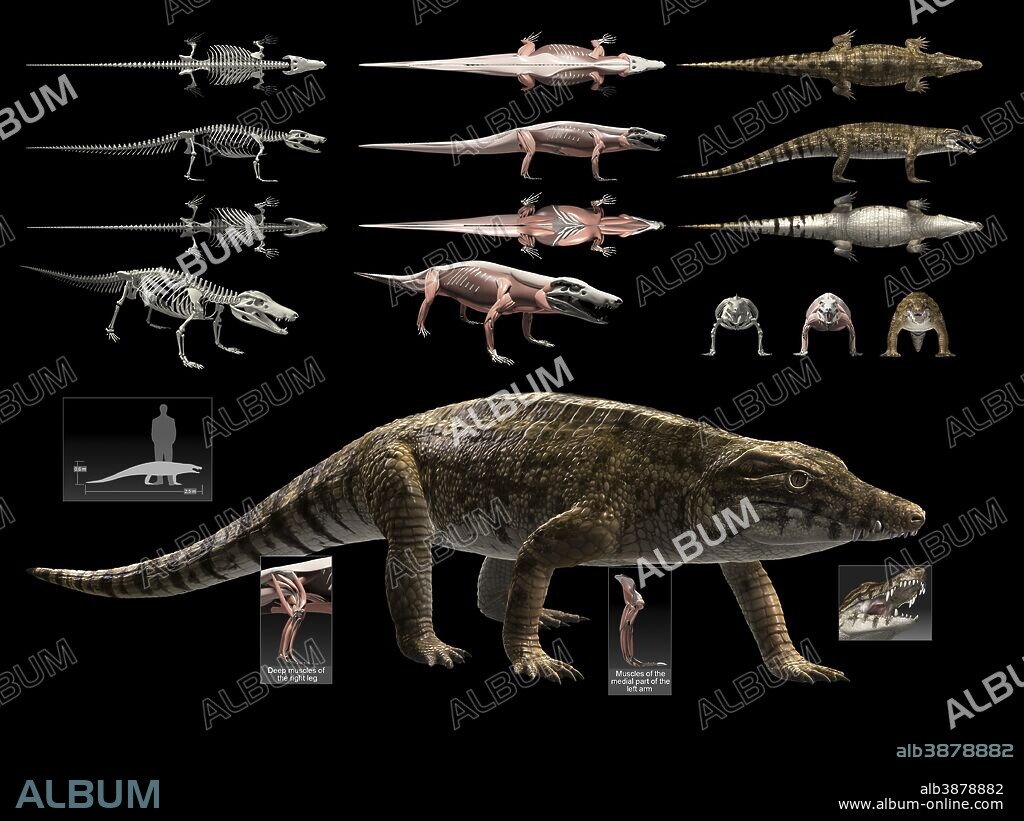This image, set against a black background, presents a detailed, multi-angle study of a green and black alligator, combined with photographic and illustrative elements. The overall display is divided into three vertical columns. The first column on the left features white illustrations of the alligator's skeletal structure, viewed from the top, side, underside, and head-on. The middle column showcases similar perspectives, but with the alligator's musculature rendered in pink, showing the skinless, detailed muscle structure. The right column depicts the alligator in its complete, natural form, displaying views from the top, side, and bottom. At the bottom center of the image, a realistic, color rendering of the alligator appears, showing it in a walking position with its nose pointing right and tail to the left. The alligator's brown scaly skin, long legs, claws, and visible eye add to the realism. Repeated across the entire graphic is a watermark that reads "ALBUM," with additional contact information and a URL "ALB3878882 www.album-online.com" in the bottom right corner. The style is a blend of photographic realism and detailed graphic design.